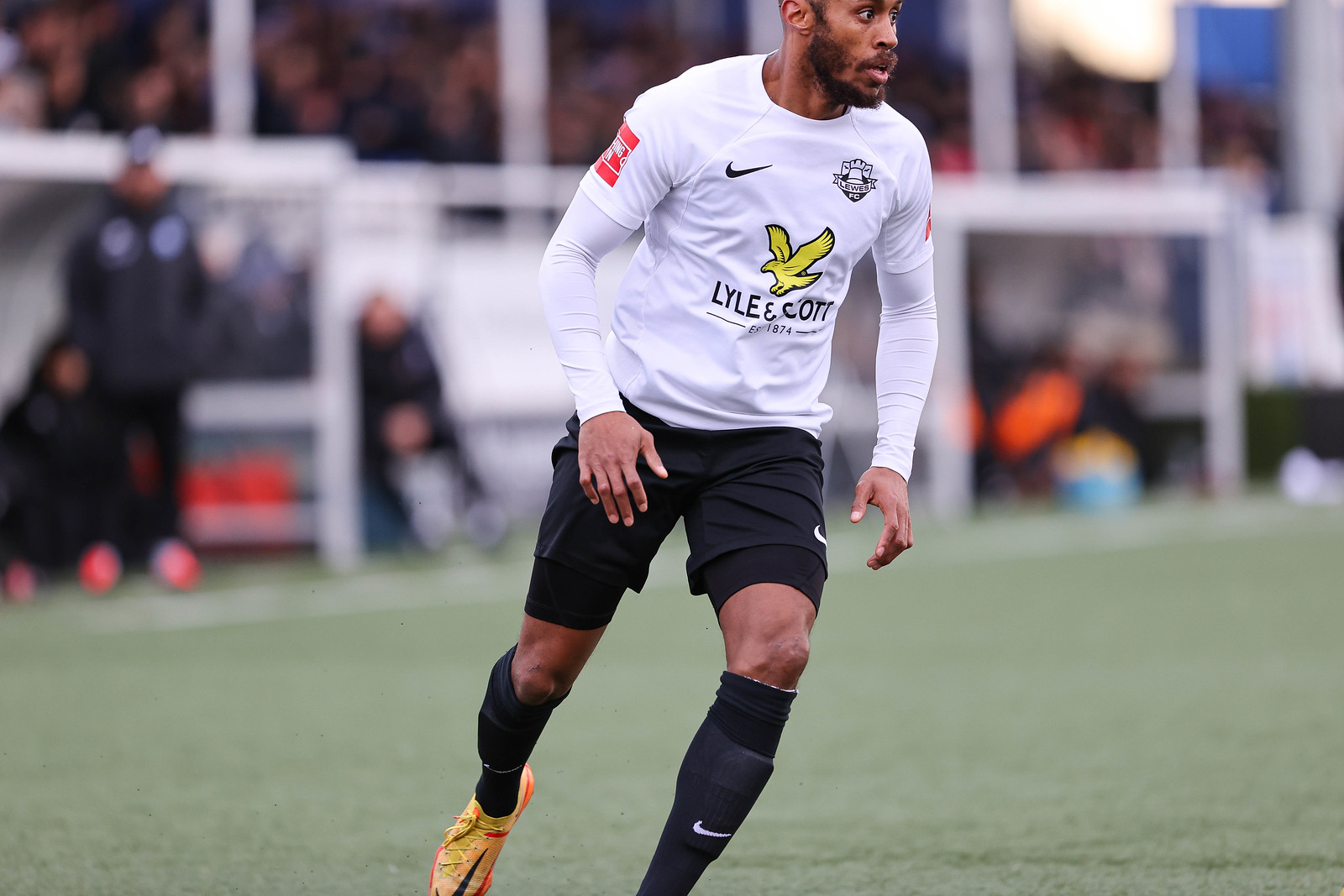In this image, we see an action shot of a black male soccer player centered on a grassy field, mid-game, with a blurred background. He is sporting a distinctive uniform consisting of a long white sleeve shirt under a short-sleeved white, yellow, orange, and black t-shirt featuring a prominent yellow bird logo and the text "Lyle & Scott, established 1874." He pairs this with black shorts revealing black compression wear underneath, black knee-high socks, and brightly colored orange and yellow cleats. The scene, captured outdoors in daylight, includes spectators in the blurry background, as well as various objects such as windows, doors, bleachers, and some people along the sidelines, including a few sitting on benches with supplies nearby. The image has a lively stadium atmosphere, emphasizing the player's dynamic presence on this well-kept soccer field.